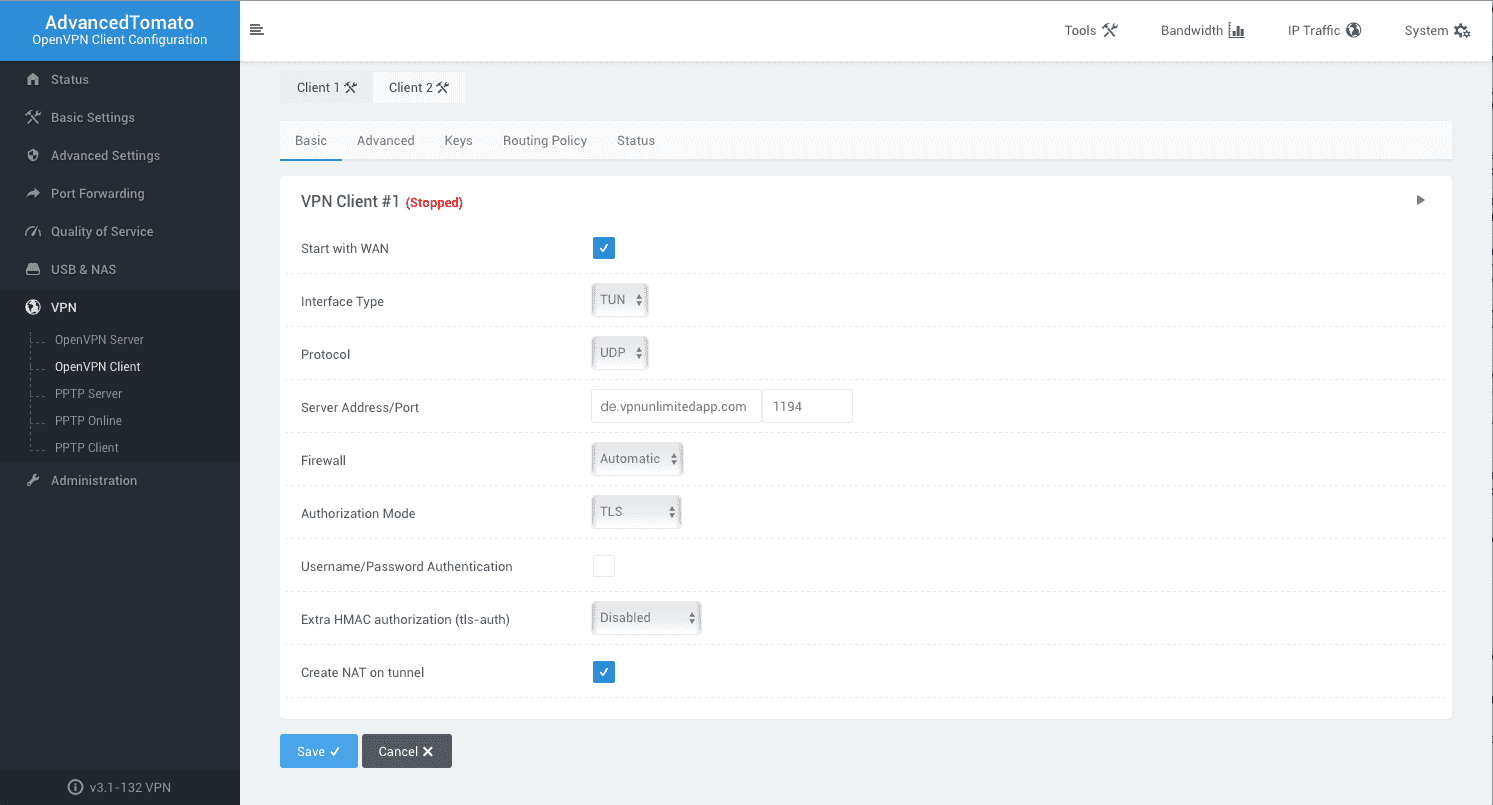The interface presented on a gray background displays the configuration settings for two clients, labeled "Client One" and "Client Two." At the top, the interface menu includes options for "Tools," "Bandwidth," "IP Traffic," and "System." Below this menu, there are two labeled keys, "Basic" and the underlined "Advanced," both highlighted in blue.

Key configuration sections are named "Routing Policy" and "Status." The VPN section is titled "Client One" denoted with a '#' symbol, and begins with the term "WAN" (Wide Area Network), which is capitalized. There is a checkbox next to it, which is currently checked. 

Further details include the "Interface Type," listed as "TUN," and another labeled section starting with the letter 'P,' suggesting it is possibly "Protocol" or a related term, accompanied by the abbreviation "LDP." This section also features fields for "Server Address/Port" that resemble a website URL format.

Other configuration parameters include "Firewall," set to "Automatic," and "Authorization Mode," set to "TLS." There are sections for "Username/Password" and "Username/Password Authentication," both with checkboxes that are not checked at present. At the bottom, the interface contains two buttons: a blue rectangle labeled "Save," and a gray rectangle labeled "Cancel."